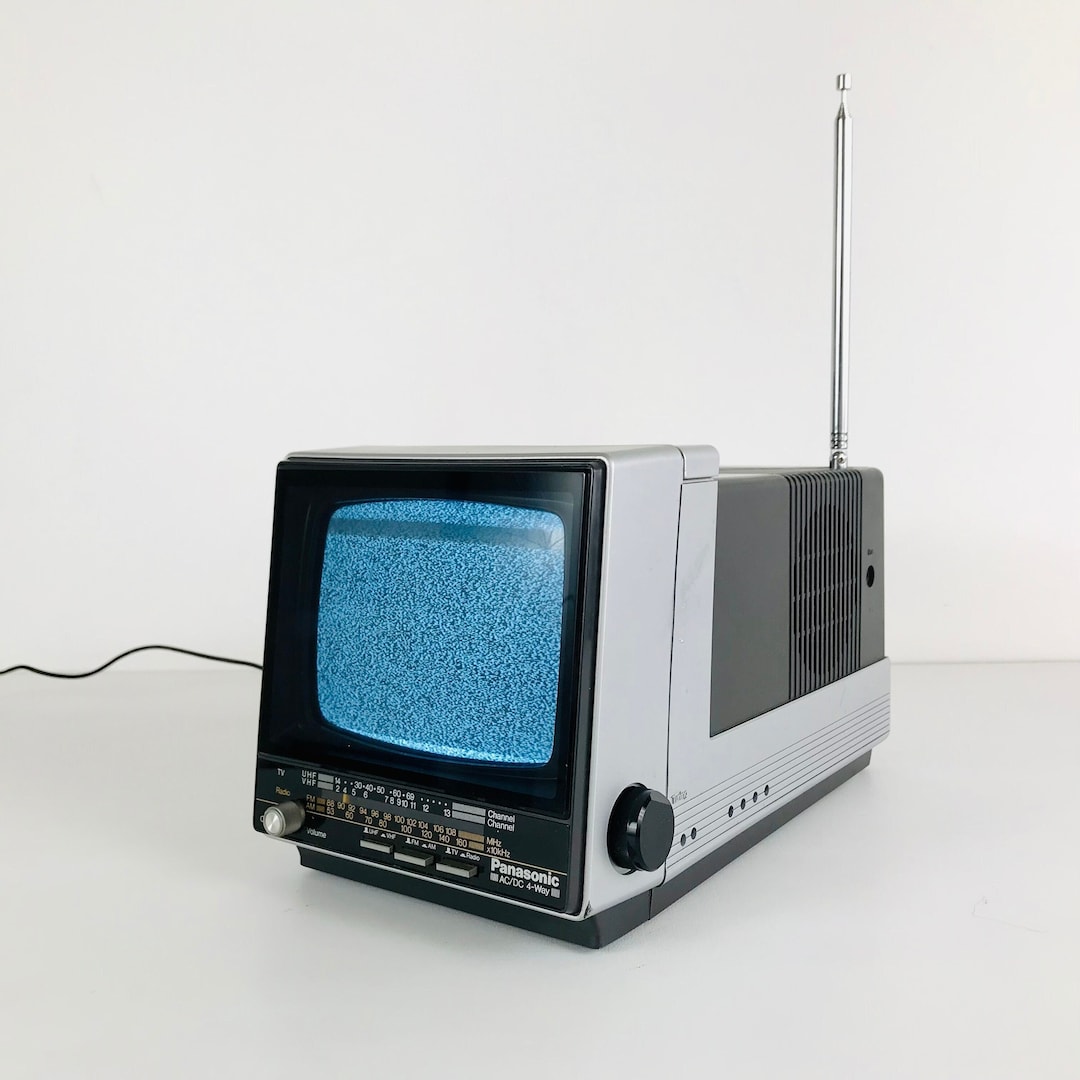This photograph showcases a vintage Panasonic color television set, accented in light gray and dark gray plastic with a black front panel. The compact TV features a square screen displaying a blue and white static pattern against a white table and wall backdrop. Prominently, the front panel bears the Panasonic logo and indicates "AC-DC" and "four-way" functionality. Below the screen lies an array of controls: a large tuning knob on the left, flanked by three flat, rectangular buttons. To the right of these buttons is a display showing radio station frequencies ranging up to the 150s. The right side of the TV houses a large black knob for additional adjustments and six adapter holes. Atop the set, a swiveling silver metal antenna stands upright. The black power cable partly visible at the back completes this nostalgic piece of electronic equipment.